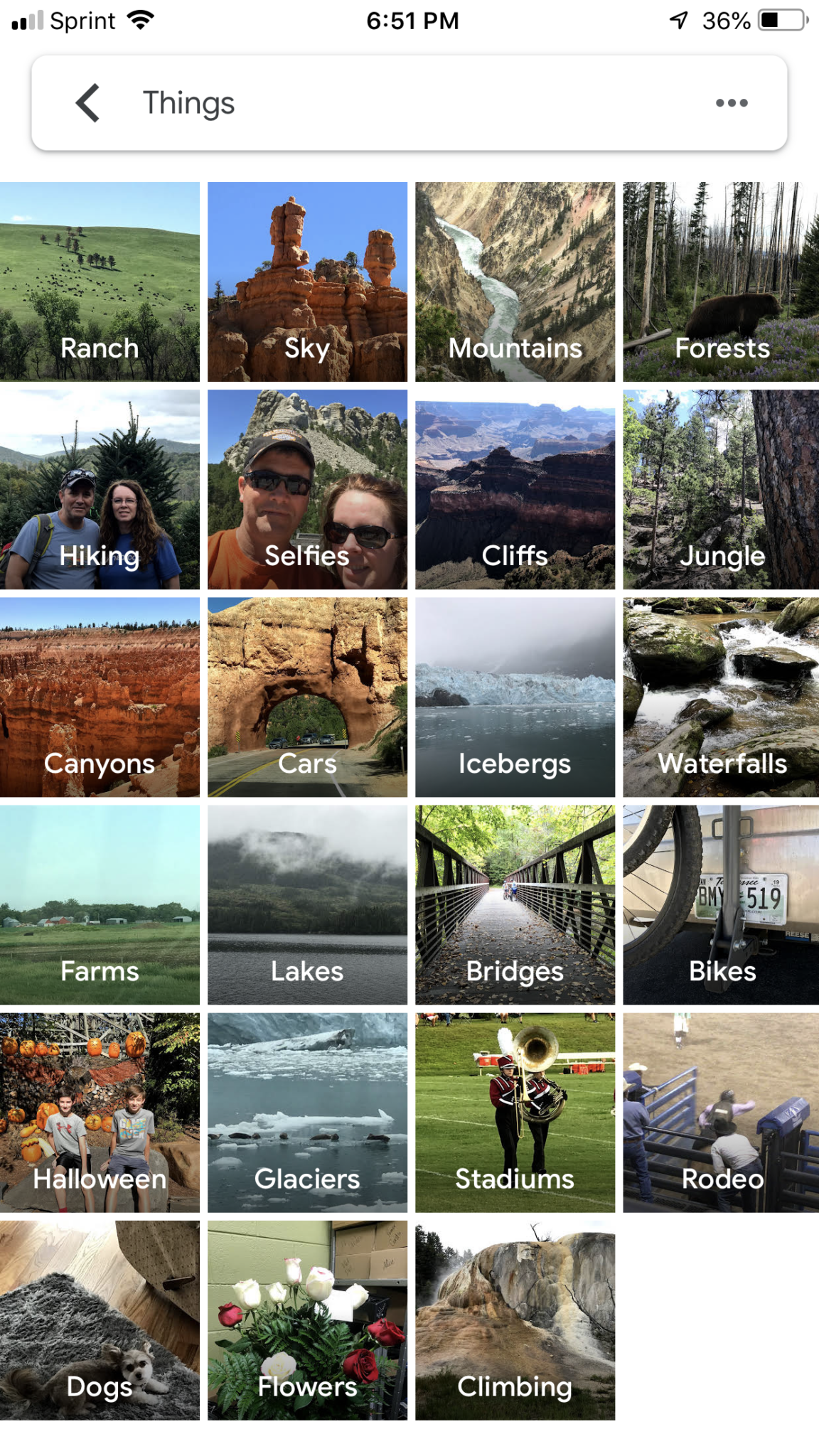The image depicts a smartphone screenshot with dimensions approximately 2 to 2.5 times taller than it is wide. It features a white background. In the top left corner, the display shows a wireless signal strength of 2 out of 4 bars next to the carrier name "Sprint," followed by full cellular signal bars. Centrally located is the time, 6:51 p.m. In the top right corner, the battery status is indicated to be at 36%.

Below this information, there is a horizontal, rounded-edged rectangle with a left-pointing black arrow on the far left. Adjacent to the arrow, the word "Things" is written in black text. On the far right of the rectangle, there are three horizontal dots.

Beneath this section, the main content is a grid layout comprising various themes and locations, arranged in a 4x6 grid. The very last cell of the grid is blank, making it a total of 23 filled cells. Each cell contains an image with corresponding descriptive text in white at the bottom. The themes include Ranch, Sky, Mountains, Forests, Hiking, Selfies, Cliffs, Jungle, Canyons, Cars, Icebergs, Waterfalls, Farms, Lakes, Bridges, Bikes, Halloween, Glaciers, Stadiums, Rodeo, Dogs, Flowers, and Climbing.